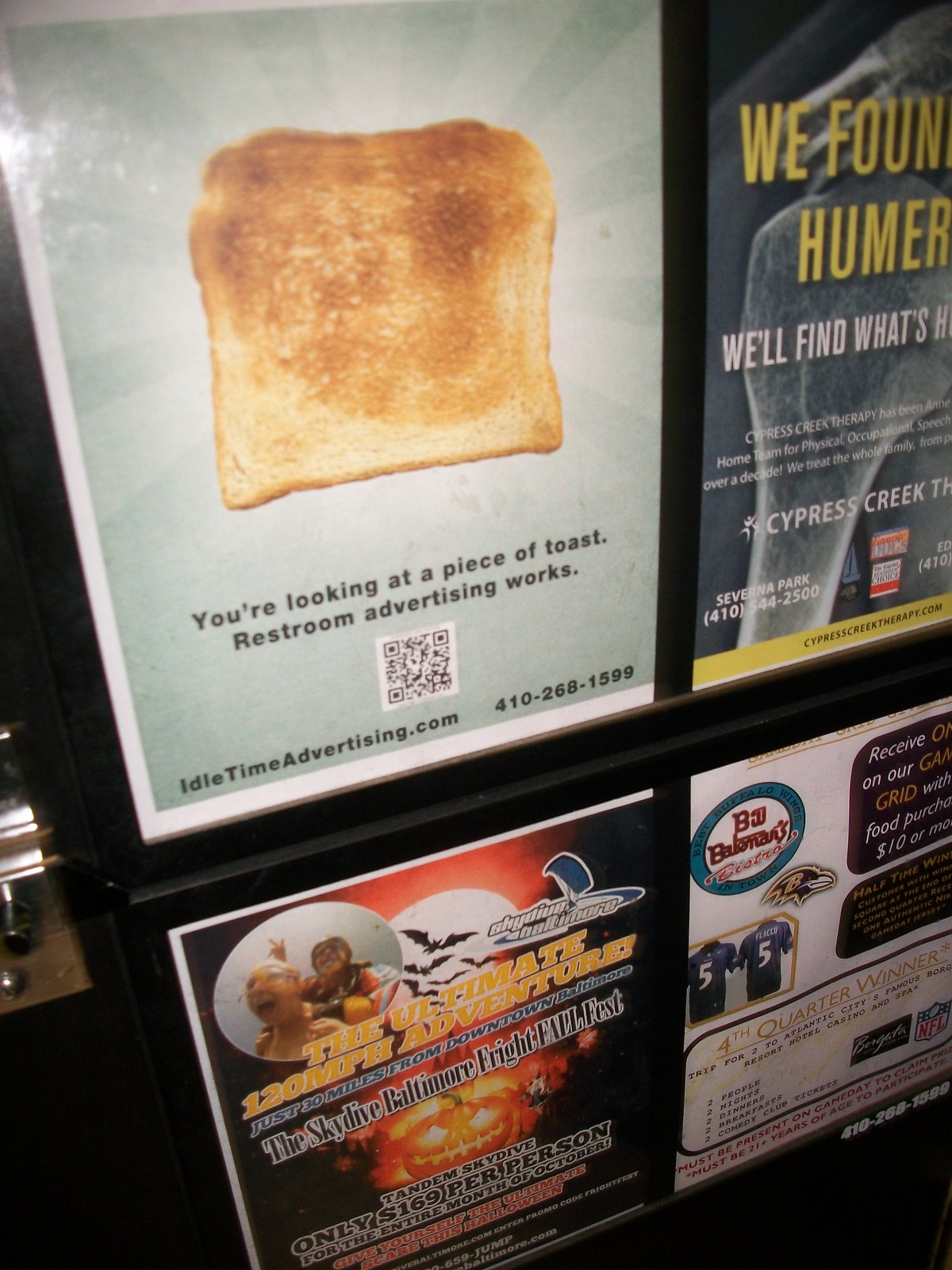The image depicts a black-framed advertisement board in a restroom, showcasing four distinct ads. The upper left quadrant features a lightly toasted piece of bread with the caption "You're looking at a piece of toast. Restroom advertising works." Below this is a QR code and the website idletimeadvertising.com, along with the phone number 410-268-1599. Beside it, on the upper right, there's an ad promoting Cypress Creek Therapy, partially visible with the phrase "We'll find what's...". The lower left section advertises a skydiving experience with Halloween-themed imagery, including pumpkins and bats, stating "The ultimate 120 miles per hour adventure. Just 30 miles from downtown Baltimore. Skydive Baltimore Fright Fall Fest." Finally, the lower right ad showcases logos of the Baltimore Ravens and the NFL, promoting BJ Batomar's Bistro.